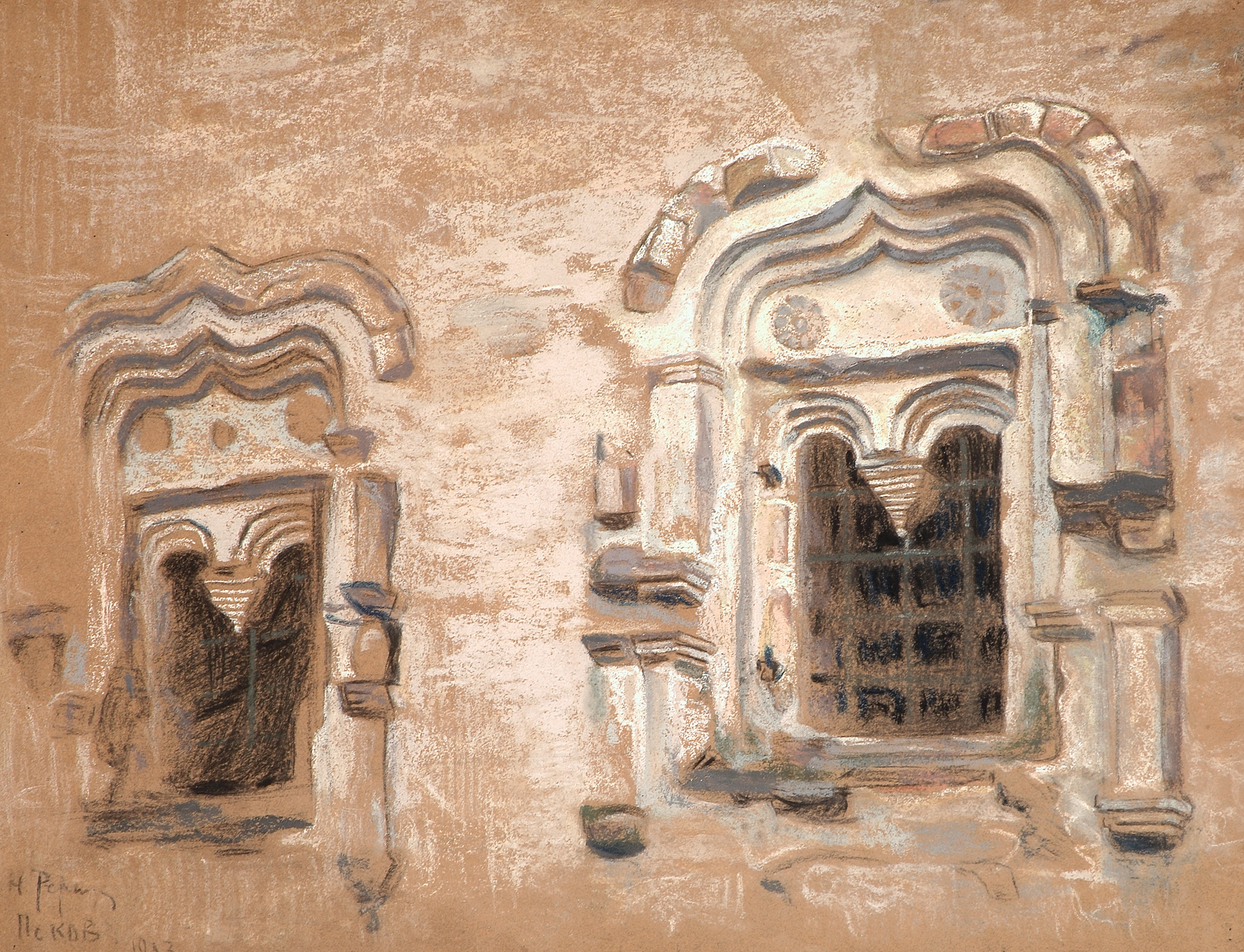The painting showcases two intricately designed windows embedded in a light brown, clay-like wall, emphasizing a Middle Eastern or Arabic architectural style. The artist employs dots from the brush, lending a rough surface effect to the wall, and a somewhat grainy, scratched texture. The smaller window on the left features a unique three-sided arch with a wavy top and a central triangle, transitioning into layered background detailing. Below it, a little rectangle section with tiny brown dots marks the top left and right sides, leading to two small meeting arches in the middle, crowned with an inverted triangle and a blackish colored inner section. The larger window on the right mirrors the overall style but is slightly broader and framed with a brick-like arch adorned with an iron gate. Both windows have deeply carved, layered frames, adding to their ornate appearance and creating an impression of depth. The bottom left of the painting bears the artist's signature, albeit indistinct. The composition, possibly rendered in acrylic with a chalky effect, captures the essence of deserty hues and white accents, encapsulating the ambiance of the subject.